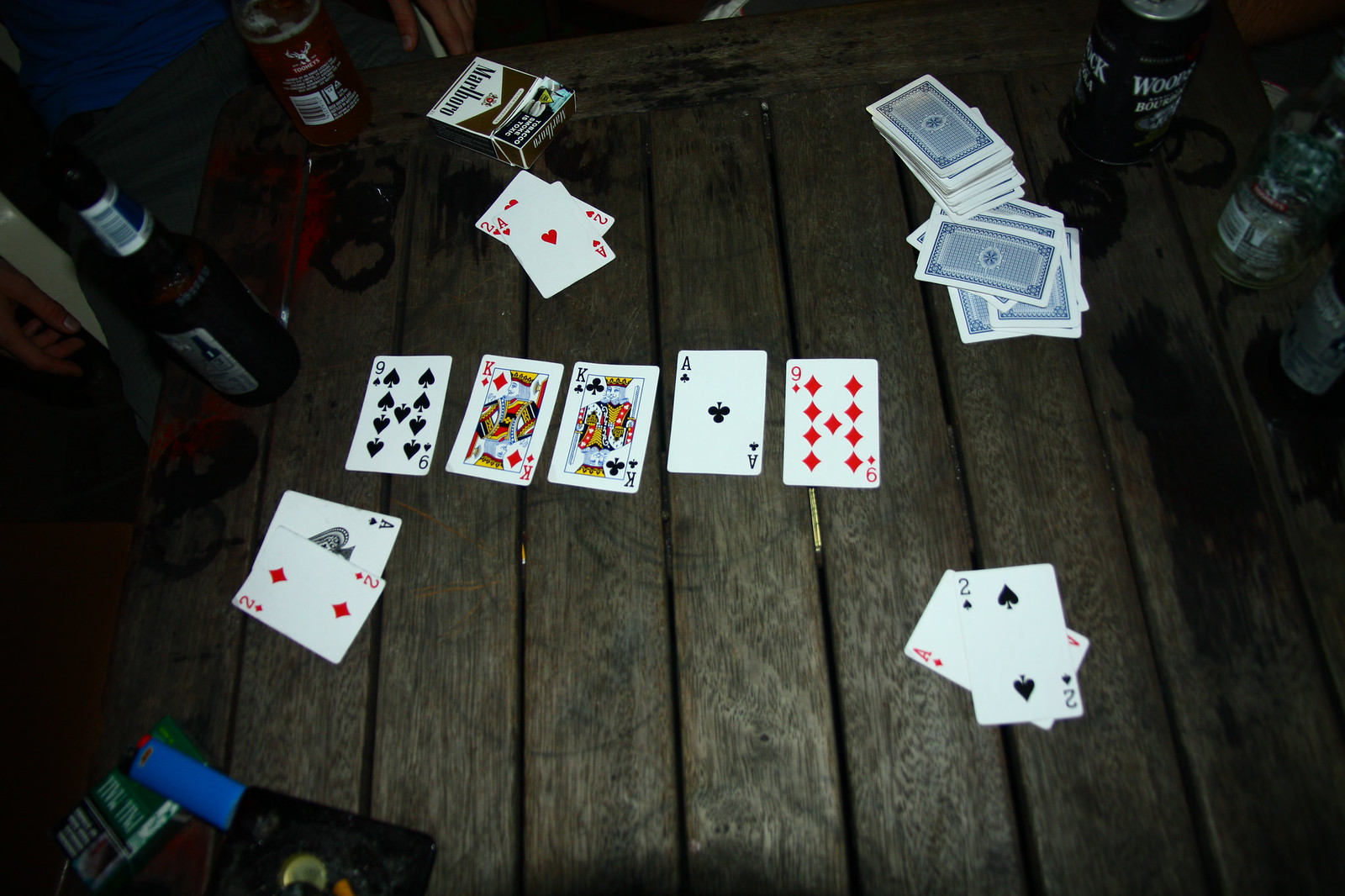This vibrant snapshot, taken from an overhead perspective with artificial lighting, captures a lively scene of friends gathered for a poker night. At the center of the image, a line of five playing cards is prominently displayed; two of these cards are kings, hinting at an arrangement for a game of poker. Alongside the main line of cards are three additional piles, two cards each, likely part of the game in progress. To the right, a disheveled pile of cards adds a casual, spontaneous touch to the tableau.

Encircling the cards are several beer bottles, each testament to the laid-back, convivial atmosphere of the gathering. A pack of cigarettes and a blue lighter sit nearby, adding to the scene’s authenticity. The cards and bottles rest on a porch or slatted floor, with dark sienna-brown floorboards set apart by narrow gaps. The floor bears a few spills, possibly from beer, enhancing the informal, carefree vibe of the evening. Despite the mess, the photograph captures the heart of the poker game, painting a vivid picture of a night filled with camaraderie and leisure.